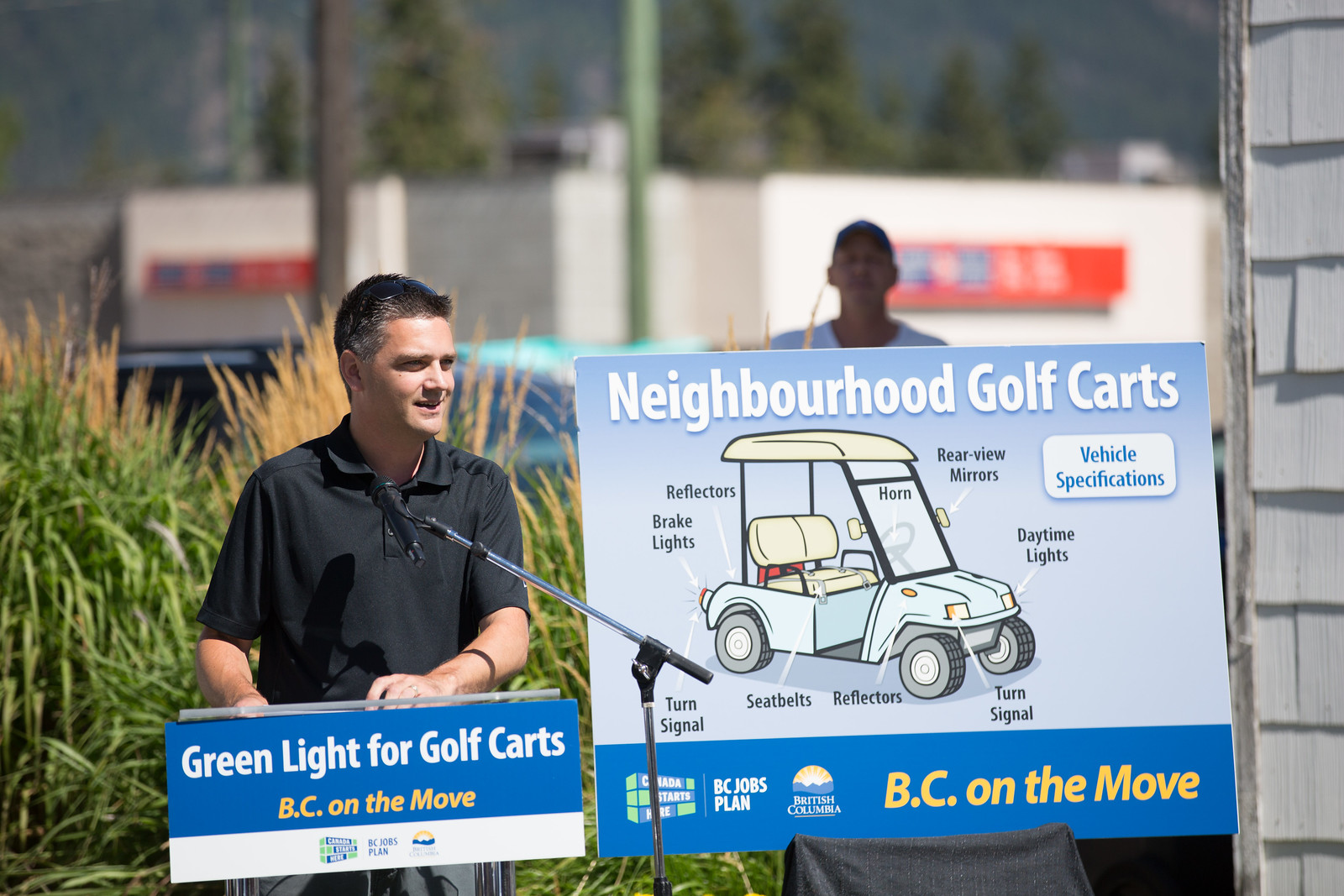This full-color photograph depicts an outdoor event under sunny and pleasant weather conditions. The backdrop features fuzzy images of trees, telephone poles, semi-trucks, and vaguely visible stores in the distance. A person in a white t-shirt can be seen in the background, but the foreground is dominated by a man, likely in his 40s, with graying hair, dressed in a black short-sleeved polo shirt. He is standing at a podium with his hands resting on it, looking off to his left with a smile on his face, illuminated by the sunlight. The podium in front of him bears a sign with the text "Green Light for Golf Carts" in blue, followed by "BC on the move" in orange. To his left, there is a larger poster labeled "Neighborhood Golf Carts," featuring a detailed diagram of a golf cart with labeled parts including rearview mirrors, horn, reflectors, brake lights, turn signals, seatbelts, and daytime lights. The bottom of this poster includes the "BC Jobs Plan" printed below the British Columbia logo, with another "BC on the move" in yellow on blue to the right. The setting includes tall grass predominantly green with brown tips, emphasizing the natural environment. The man speaks into a microphone, adding to the formal atmosphere of the event.